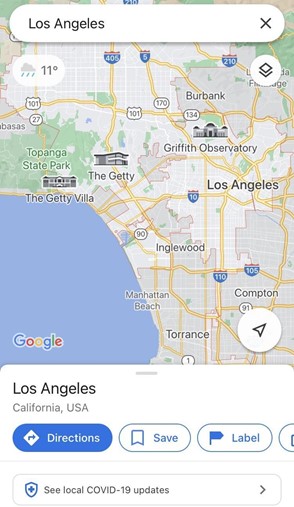This is a detailed screenshot of the Google Maps web application displaying Los Angeles, California, USA. At the top of the image is a white search bar stretching across the full width of the screen. Within this bar, the text "Los Angeles" is visible in black, along with an "X" icon on the right to close the search. Directly below, on the left side, is a smaller bubble displaying the current weather: an 11 degrees icon beside a rain cloud symbol with three diagonal rain lines. Below the “X” icon, there is a layers button resembling a diamond with an outline at its base for adjusting the map view.

The map of Los Angeles features various neighborhoods shaded light gray and outlined in orange. Three significant landmarks are marked on the map: 
1. The Getty Villa, depicted with an icon that resembles a colonial-style villa, located below Topanga State Park.
2. The Getty Center, represented by a modern building icon, situated to the northeast of the Getty Villa.
3. The Griffith Observatory, illustrated with an icon resembling a political capitol building, positioned further northeast of The Getty Center.

Additionally, several other city names are visible on the map, including Burbank, Inglewood, Compton, Torrance, and Manhattan Beach. 

At the bottom left corner, the Google brand name is discernible, while at the bottom right corner, there's a navigation compass inside a white circle. Along the bottom of the image, text indicates the location as "Los Angeles, California, USA," accompanied by action buttons for directions (featuring a street sign symbol), saving (depicted by a save banner icon), and labeling (shown with a blue flag). Below these buttons, a gray dividing line separates a box containing the text "See local COVID-19 updates," complete with a shield and a medical plus symbol, and an arrow to expand the box for more information.